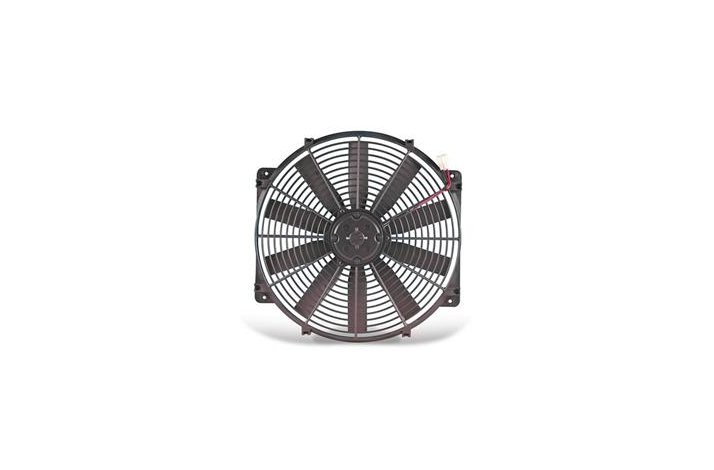This image features a large fan against a white background. The primarily black or dark gray fan is circular with ten thin blades radiating from a central hub. The blades are protected by a circular grill, which is likely dark metal gray, preventing any hands from accidentally touching them. The fan is equipped with a square mounting bracket on each side with four screw holes, suggesting it can be securely attached to various devices, potentially a computer case or a car radiator. Notably, in the top right corner of the image, a pair of wires—one red and the other possibly green or black—extend upwards and to the right, terminating in a small white connector that indicates it can be plugged into a DC power source. The fan gives an impression of multi-use, industrial capability, and is detailed with shadows underlining the fan on the otherwise plain white backdrop.